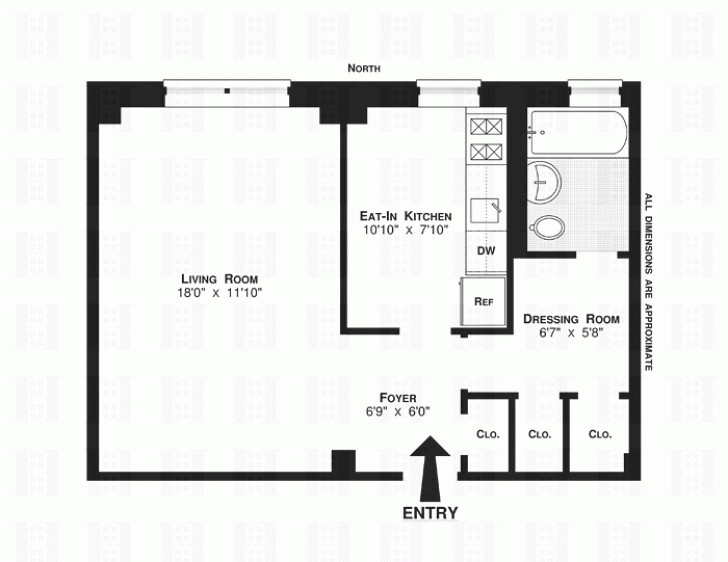This detailed blueprint depicts a ground-level apartment layout against a black background or border. On the right side, the caption "All dimensions are approximate" is written in black letters. 

At the top of the blueprint, labeled "North," are three windows that illuminate the living room, which measures 18 feet by 11 feet 10 inches. Adjacent to the living room is a foyer measuring 6 feet 9 inches by 6 feet. 

The main entry is indicated by a black arrow situated at the bottom of the layout. Upon entering, there's a closet on one side, followed by two additional closets and a dressing room measuring 6 feet 7 inches by 5 feet 8 inches. This dressing room leads into the bathroom, which is equipped with a toilet, sink, and bathtub, along with a window for ventilation.

The eat-in kitchen measures 10 feet 10 inches by 7 feet 10 inches and features essential appliances such as a refrigerator, dishwasher, sink, and stove. The kitchen area includes four black X's marking additional windows. 

The dressing room is separated from the living room by a wall, which includes a doorway providing access between the two spaces.